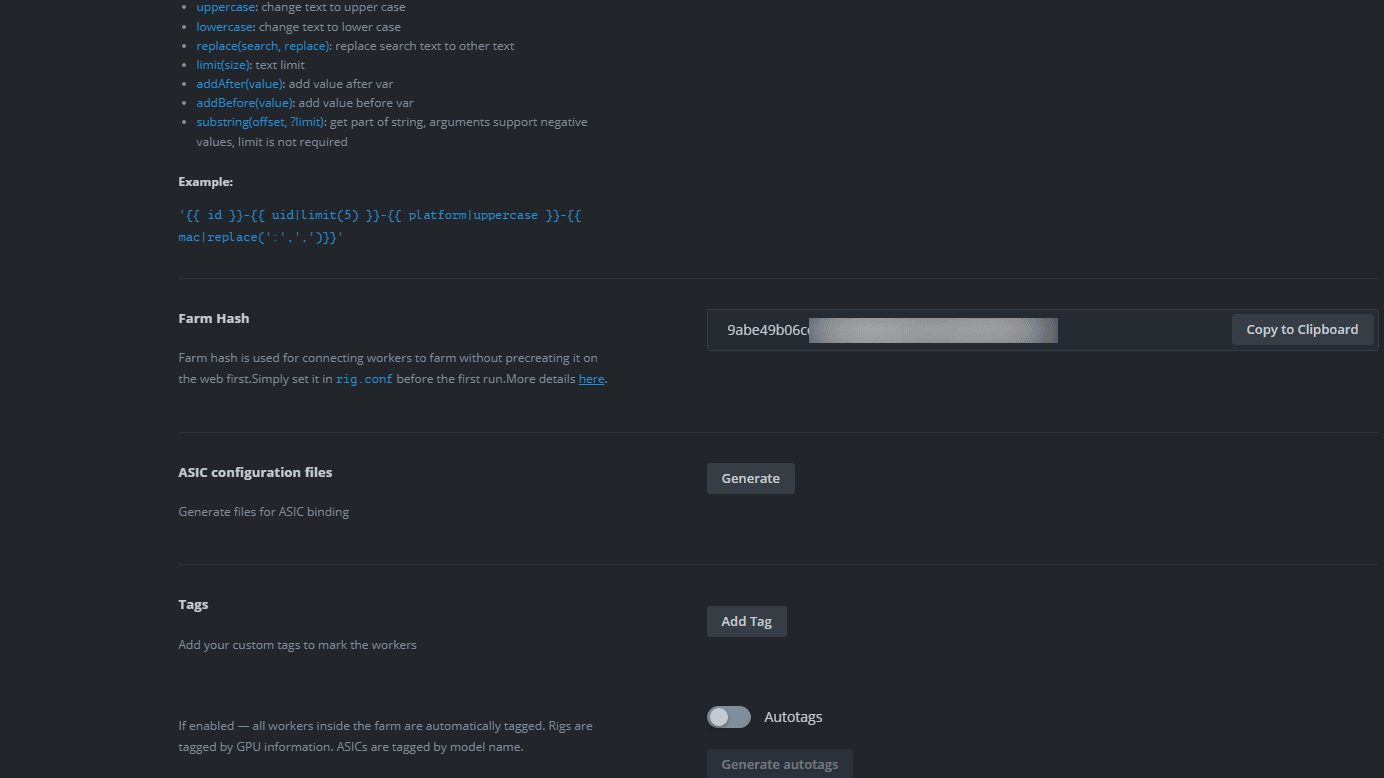This is a screenshot of a coding website interface. The interface features multiple blue, clickable links. At the top section, an example code snippet is displayed: 

```
'apostrophe [[[ID]]]] UID/LIMIT(5)[[[platform/Uppercase[[[[R-A-C-replace(':'..')]]]]]']]]. 
```

Below the code snippet, there is a detailed description stating: 

"Farm Hash: Farm Hash is used for connecting workers to a farm without presenting it on the web first. Simply set in `rig.conf` before the first run for more details."

Further down, there is a header labeled "ASIC Configuration Files," with a button below that labeled "Generate Files for ASIC Basic." At the very bottom, there is an option to add tags, accompanied by an "Add Tags" button.